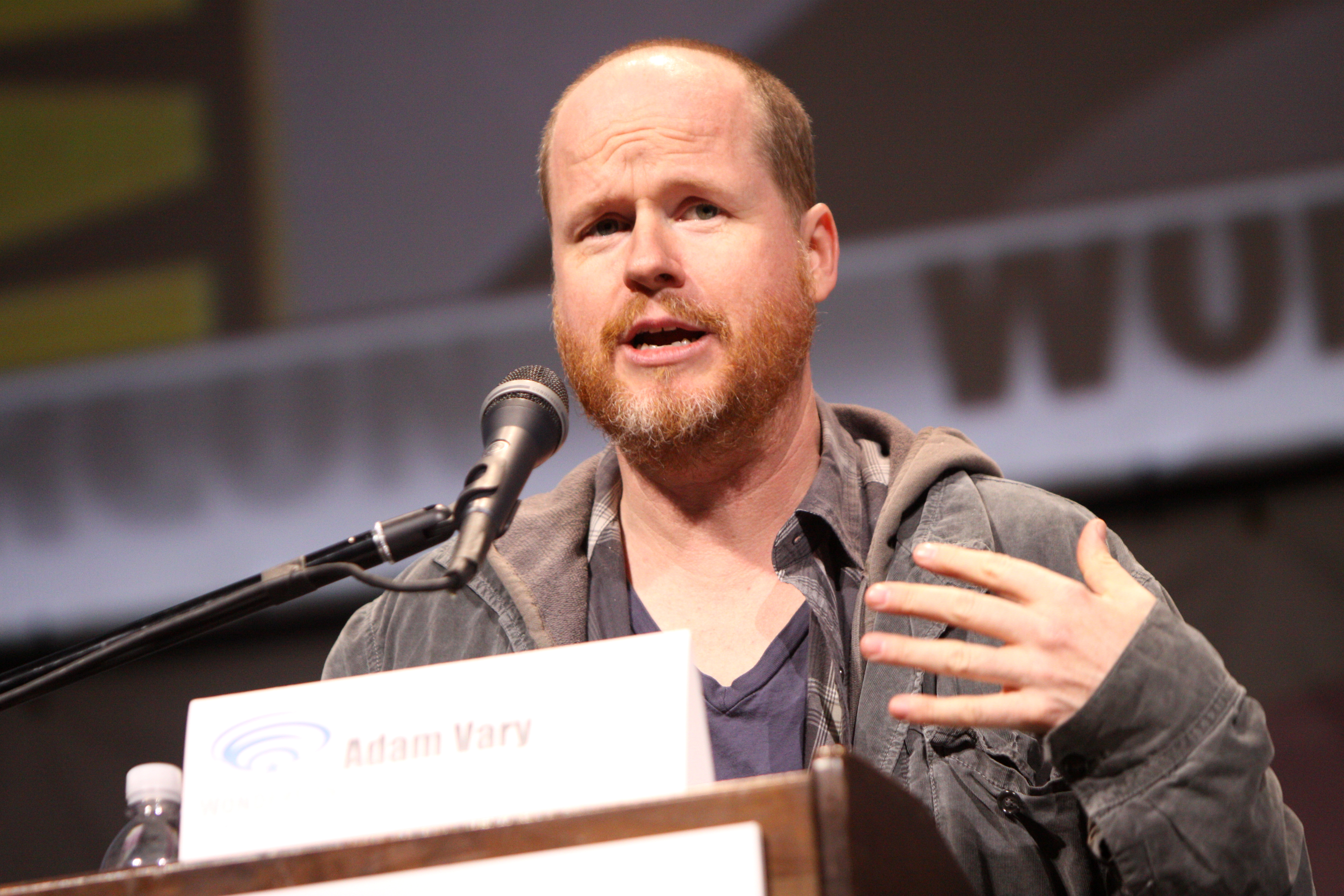The image depicts a close-up of a Caucasian man, approximately in his mid-30s to mid-40s, speaking at a wooden podium. He has a receding hairline, very short reddish hair, and a reddish-silver beard. He is dressed in a dark gray jacket with a navy blue V-neck shirt underneath. The podium bears a white name tag with the name "Adam Vary" inscribed in a dark brown sans-serif font. Positioned on the left side of the podium is a water bottle. A wired microphone, gray in color with black and silver accents, is pointed towards him. The man is seen gesturing with his hand as he speaks, and in the background, there is a blurred blend of white, gray, and yellow colors, along with partially visible black text, including the letters "WU."